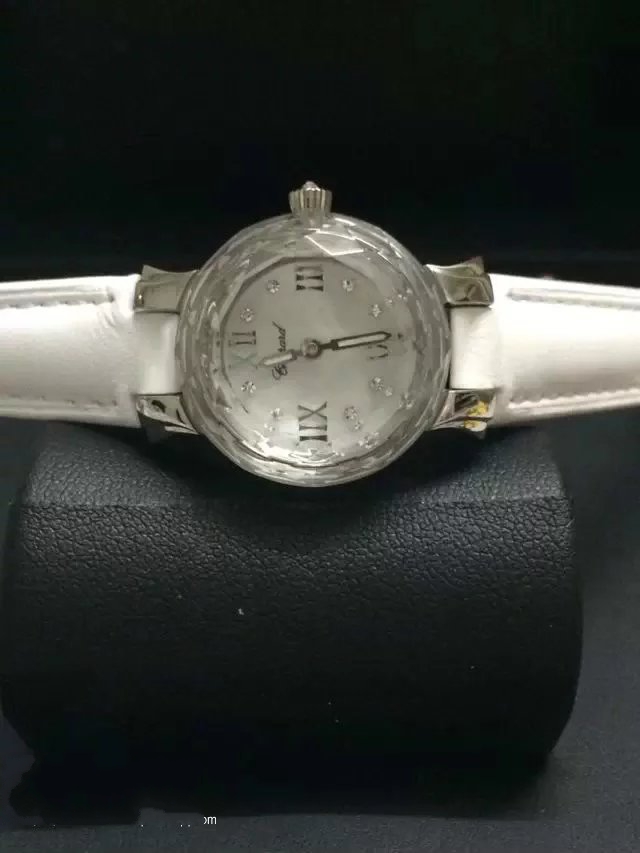An up-close, detailed photograph of a sophisticated watch, prominently displayed on a black styrofoam base that blends seamlessly with a completely black background. The watch features elegant white leather straps and a faceplate bordered by an opaque, clear material bezel. The time displayed is approximately 11:29, with the hour and minute hands nearing 12 and 6 respectively. The watch face is adorned with Roman numerals at 12, 3, 6, and 9, adding a classic touch to its design. This close-up shot highlights the intricate details and refined craftsmanship of the timepiece.